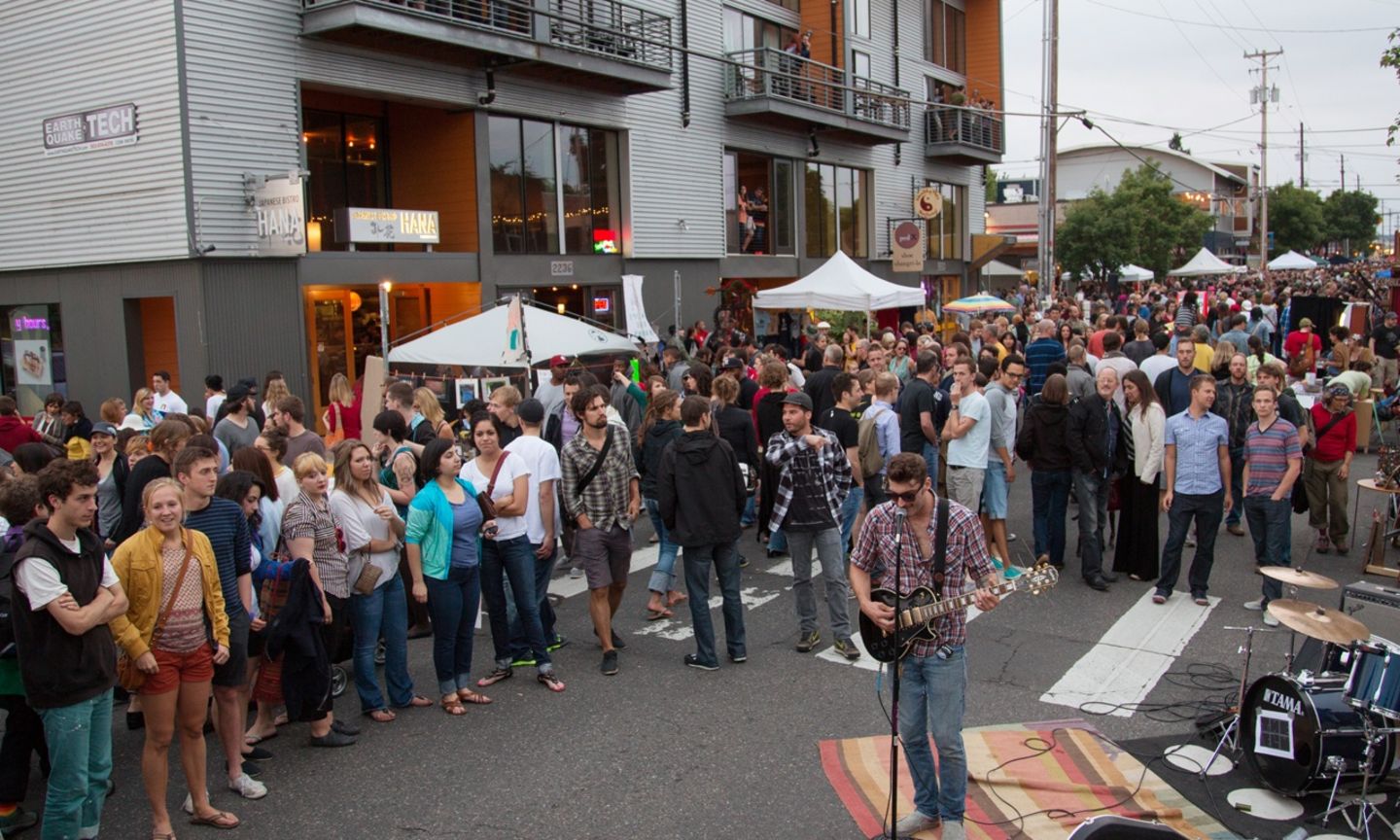The image depicts a bustling street fair or outdoor concert in a city or town. At the forefront, to the right of center, stands a man in a short-sleeved plaid shirt, jeans, and sunglasses, with medium-length brown hair. He is performing with a black guitar and singing into a microphone mounted on a stand. Beneath him is a large multicolored rug in shades of red, dark brown, orange, tan, and yellow. A black drum set is partially visible to his right. The background is alive with activity: a crowd fills the street, stretching from the foreground to the distant background, lined up shoulder to shoulder. Behind the performer, a crosswalk is visible, teeming with people. The street is adorned with white umbrellas and tents, indicating market stalls or vendor booths. On the left, the street is bordered by buildings, one with windows on the second floor and three metal terraces above, and large buildings loom in the background along with trees and power lines. The scene captures the energetic and vibrant atmosphere of the outdoor event.